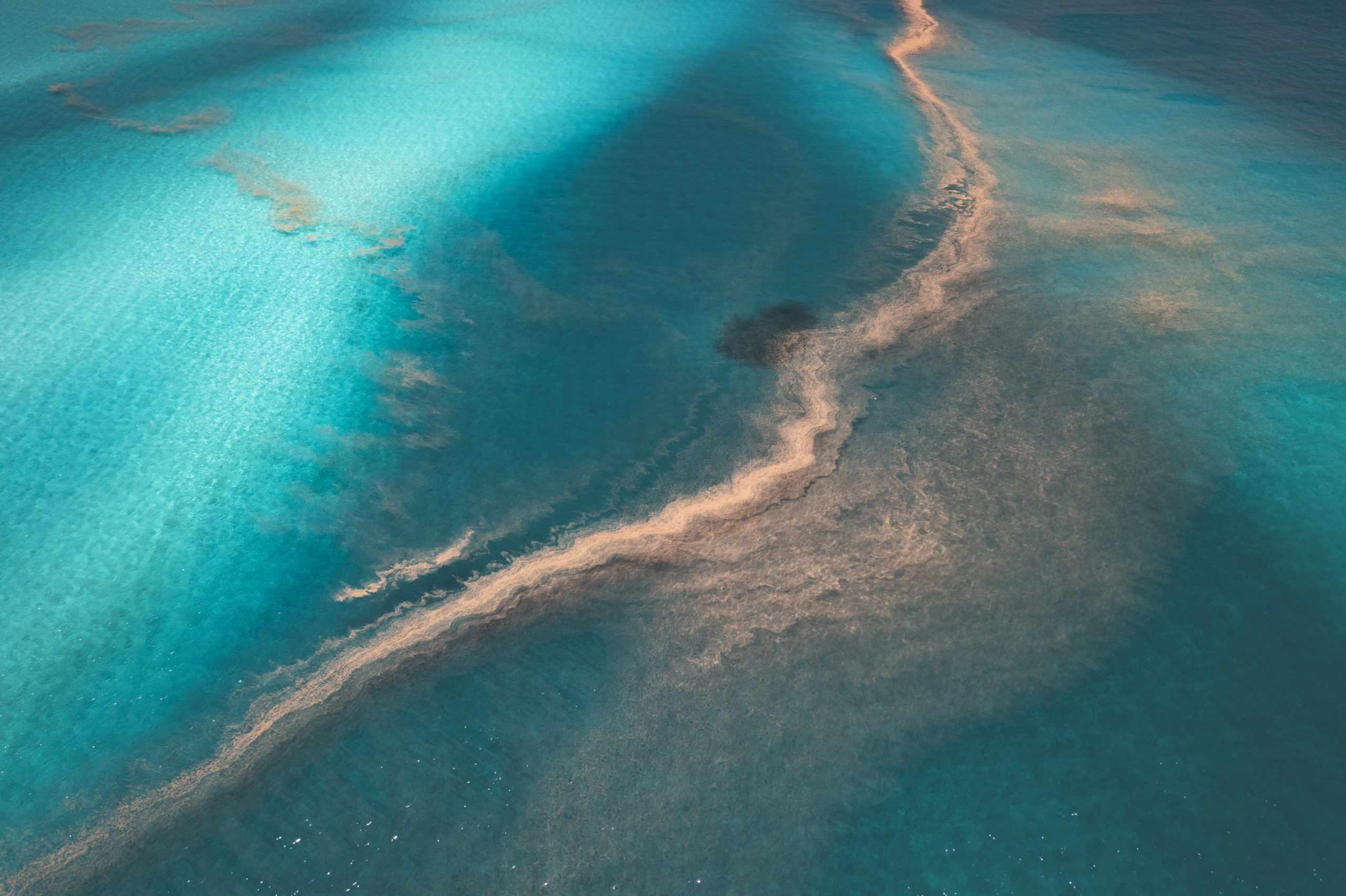This color photograph, likely taken from an airplane, captures a vast expanse of an ocean or sea from an aerial perspective. The image is dominated by water, varying from bright blue in the upper left corner to darker shades as it transitions to the right. The most striking feature is a crooked, wiggly, light brown trail running diagonally across the center, which appears to be composed of sand or perhaps some spilled material, giving the water a murky quality with brown, foamy waves. The left side of the ocean is more illuminated by sunlight, while the right side remains darker and more obscure. The overall scene conveys a sense of calmness, punctuated by faint ripples and the peculiar trail disrupting the uniformity of the vast blue expanse.